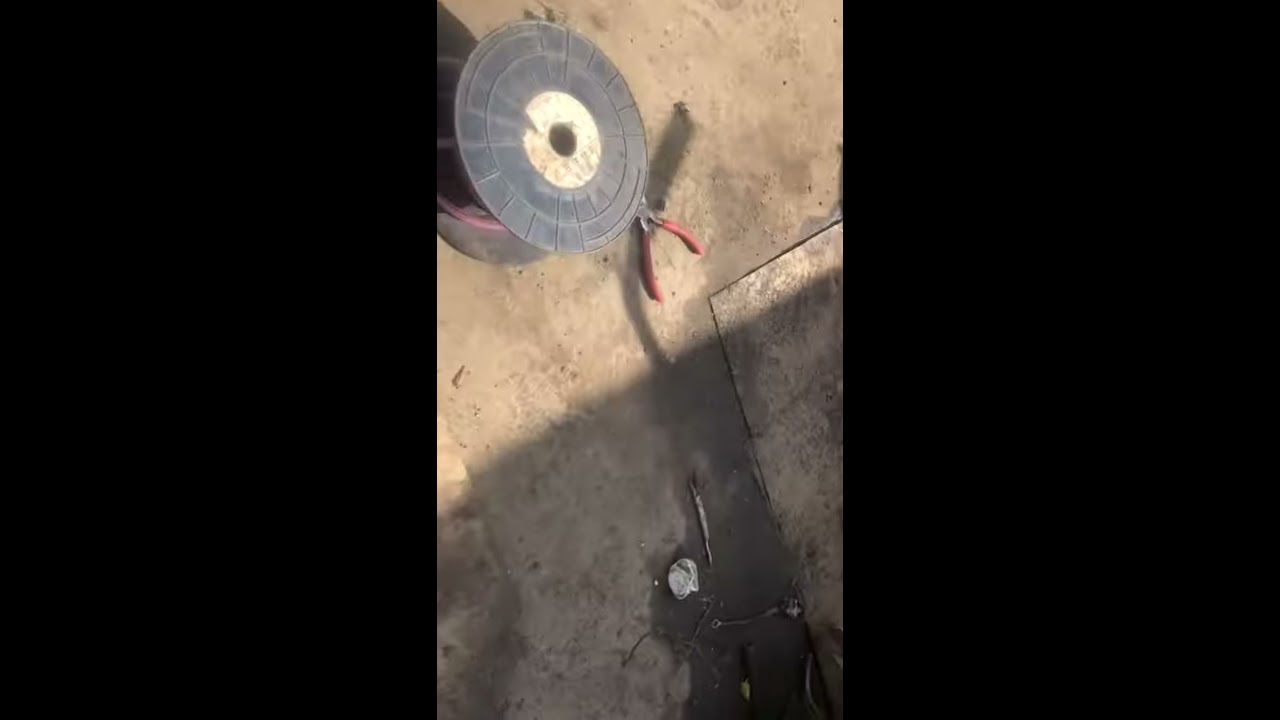The image shows a close-up view of a dirty, dusty, and stained concrete floor, likely part of a construction site. The photograph is taken from above, capturing various tools and debris scattered across the ground. In the top left corner, there's a large black plastic spool, possibly for wire or hose. To the right of this spool, near the center of the image, lies a pair of pliers with red handles. The ground itself, a brownish-gray concrete, includes some wet spots and a square indentation in the bottom right corner. Additionally, this area of the image is littered with loose wires and other small construction debris. The lighting is uneven, illuminating the upper portion while casting shadows over the bottom half, giving a sense of depth and dimension to the scene.